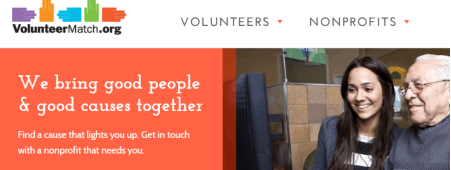This is a screenshot of a VolunteerMatch.org page. The top section features a row of colorful hands: a purple hand pointing left, an orange hand with the palm facing upwards, a blue hand with fingertips pointing right, a green hand with fingertips pointing up, and another orange hand with fingertips pointing to the right. Below this line of hands, there are two navigation options: "Volunteers" and "Nonprofits," both written in black font over a white background and accompanied by drop-down menus denoted by red triangles with their tips pointing downwards.

The left half of the page is dominated by a coral-colored box containing a message in white font: "We bring good people and good causes together. Find a cause that lights you up. Get in touch with a non-profit that needs you."

On the right side, there is a heartwarming image of a young woman and an older gentleman sitting together and looking at a computer screen to their left. The woman has long brown hair, while the gentleman, wearing glasses, has short white hair. Both are smiling, creating an inviting atmosphere. The background features a cubicle-style wall and some glass, suggesting an office environment.